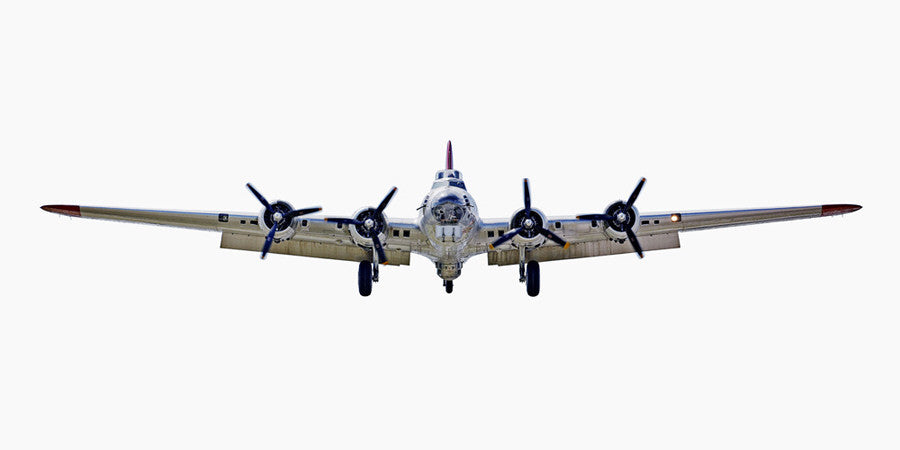This image depicts a B-17 airplane coming towards the viewer, with a white background emphasizing its presence without distraction. The large, silver jet prominently features wide wings extending on either side. Each wing supports two propeller engines, making a total of four propellers at the front. The nose of the plane has a distinct black circle, and just behind it, the pilot's compartment window is faintly visible. On the top of the airplane, a needle-shaped brown structure protrudes, likely part of the tail's silhouette. The aircraft's undercarriage displays two larger black tires at the front and a smaller one at the back. The jet’s wings also have some square black windows and maroon-tipped ends. Overall, the plane has a robust, forward-facing stance with notable details such as light fixtures on its structure.